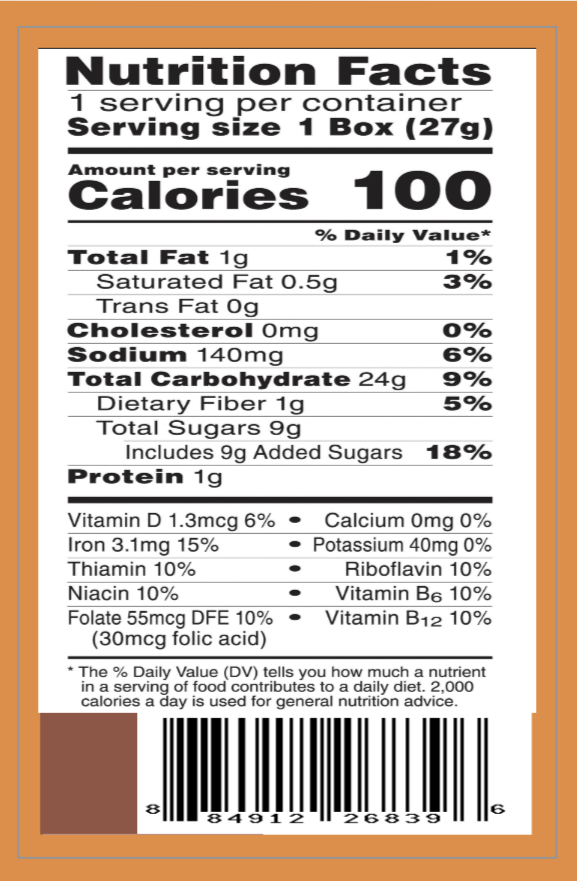The image shows a detailed Nutrition Facts label, bordered in an orangey-brown color, with the inside section featuring white background and black text. The top of the label prominently reads "Nutrition Facts." Below that, it states that there is one serving per container and that the serving size is one box (27 grams).

A black line divides this section from the next. Here, the nutritional information begins with "Amount per serving," listing calories as 100 and providing the percent daily values (%DV) for various nutrients. The breakdown is as follows:
- Total Fat: 1 gram (1% DV)
- Saturated Fat: 0.5 grams (3% DV)
- Trans Fat: 0 grams
- Cholesterol: 0 milligrams (0% DV)
- Sodium: 140 milligrams (6% DV)
- Total Carbohydrate: 24 grams (9% DV)
- Dietary Fiber: 1 gram (5% DV)
- Total Sugars: 9 grams, which includes 9 grams of added sugars (18% DV)
- Protein: 1 gram

Another black line divides this section from the lower portion, which provides information on micronutrients:
- Vitamin D: 1.3 micrograms (6% DV)
- Calcium: 0 milligrams (0% DV)
- Iron: 3.1 milligrams (15% DV)
- Potassium: 40 milligrams (0% DV)
- Thiamin: 10% DV
- Riboflavin: 10% DV
- Niacin: 10% DV
- Vitamin B6: 10% DV
- Folate: 55 micrograms DFE (10% DV), including 30 micrograms of folic acid
- Vitamin B12: 10% DV

At the bottom of the label, there's an explanation that the percent daily value (DV) indicates how much a nutrient in a serving of food contributes to a daily diet, and that 2,000 calories a day is used for general nutrition advice. Beneath this text, there is a barcode.

This comprehensive label provides all essential nutritional information in a clear and detailed manner.